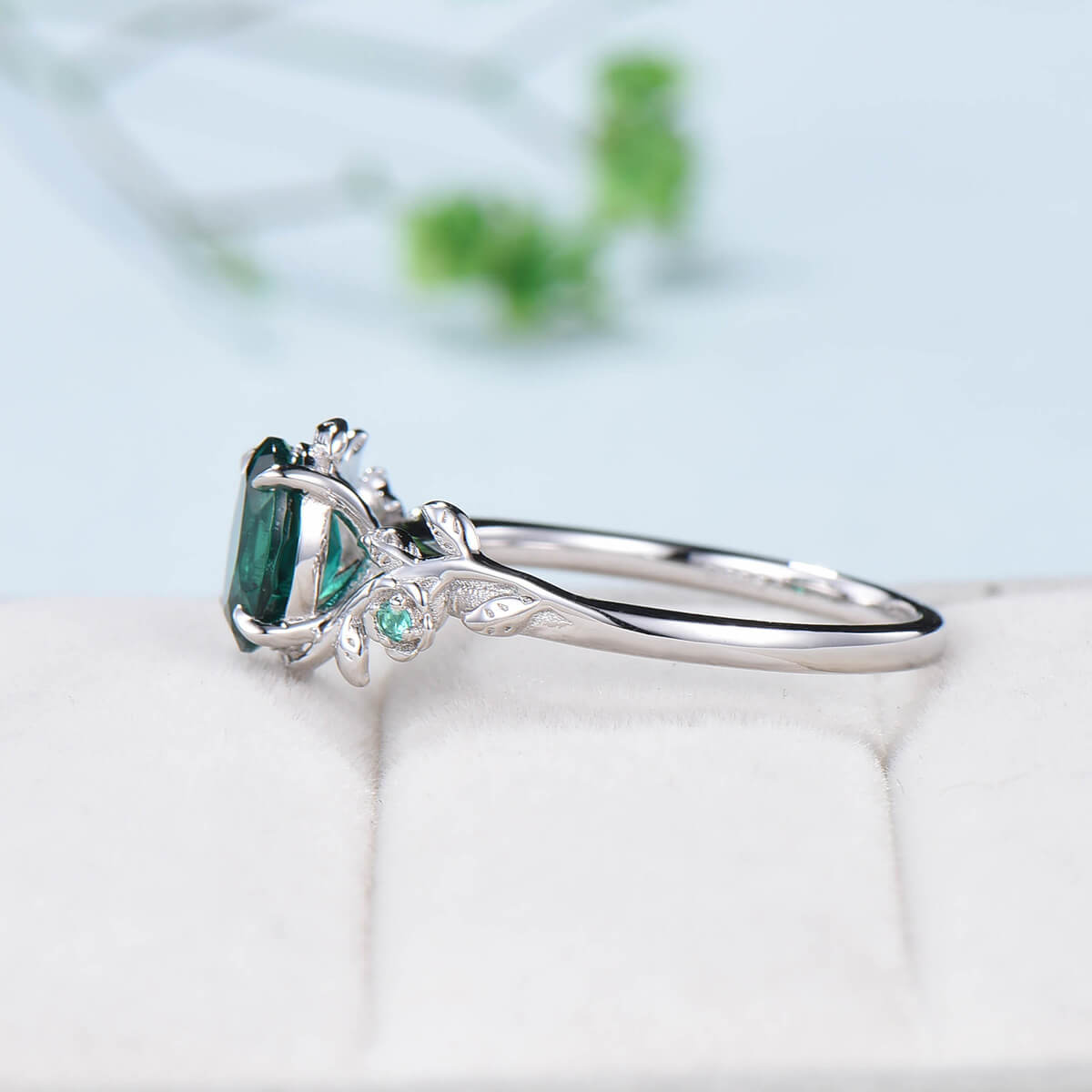A photograph showcases an elegantly crafted silver ring laid flat on a pristine, cushioned white cloth. The ring is positioned with meticulous care, emphasizing its intricate details. In the upper background, a blur of lush green leaves contrasts subtly against a light blue and white backdrop.

The centerpiece of the ring is a captivating dark green gemstone, presumably an emerald, securely held by delicately arching prongs. These prongs ascend gracefully to cradle the gemstone, ensuring a perfect fit. Along the prongs, smaller green gems and sparkling diamonds are intricately inset, adding a touch of brilliance to the sophisticated design.

The silver band itself transforms near the head of the ring, branching out into delicate, leaf-like extensions that appear to grow organically towards the central emerald. This botanical motif further enhances the ring's enchanting allure, making it a strikingly detailed and visually enchanting piece of jewelry.